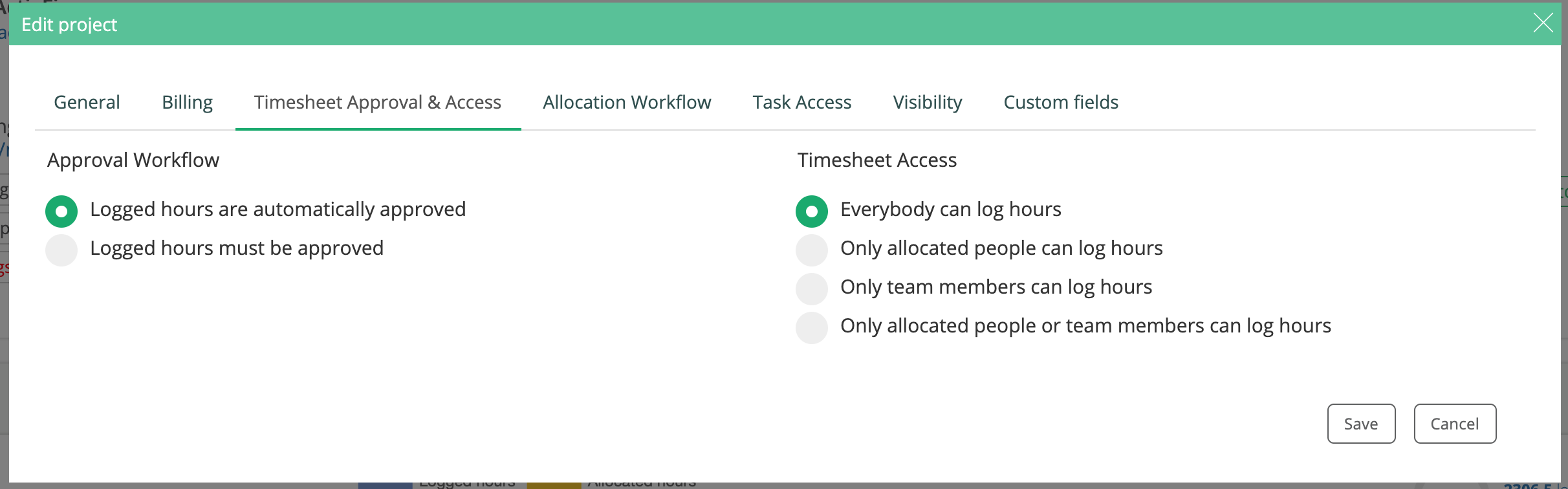The screenshot displays an interface from a project management software. The top banner is a teal color with a line containing the text “Edit Project” in white, alongside a white "X" button for closing the window. Below, there is a large white rectangle filled with black text.

At the top, there is a horizontal navigation menu consisting of sections labeled “General,” “Billing,” “Timesheet,” “Approval,” “Access,” “Allocation,” “Workflow,” “Task,” “Access,” “Visibility,” and “Custom Fields,” with a green underline indicating the selected section.

Under the “Approval” section to the left, there is a sub-section titled “Approval Workflow,” presenting two options. The first, “Logged hours are automatically approved,” is marked with a selected green circle. The second, “Logged Hours Must Be Approved,” has an unselected gray circle.

To the right, under “Timesheet Access,” there are several options for logging hours:
- "Everybody can log hours," which is selected and marked with a green circle.
- "Only Allocated People Can Log Hours," "Only Team Members Can Log Hours," and "Only Allocated People or Team Members Can Log Hours," all of which are unselected and denoted by gray circles.

At the bottom right corner of the interface, there are “Save” and “Cancel” buttons for confirming or discarding the changes.